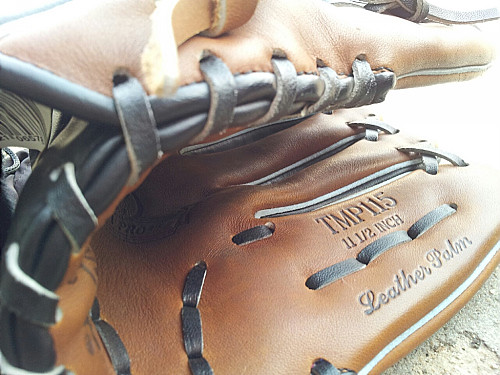This close-up color photograph zooms in on a medium brown leather baseball glove, emphasizing its detailed craftsmanship. The glove, likely new given its smooth texture, displays the text "TMP-115, 11 1/2 inch, leather palm" prominently. Black leather straps and stitching provide a striking contrast along the edges and fingers. The glove’s opening faces the camera, revealing meticulous lacing and stitching. The background is almost completely blurred out due to high brightness, though some rough, concrete-like texture is faintly visible in the lower right corner, hinting at an outdoor setting. The image, with a washed-out appearance, conveys a sense of nostalgia for a sunny day of baseball, making it an evocative marketing shot for a premium baseball glove.